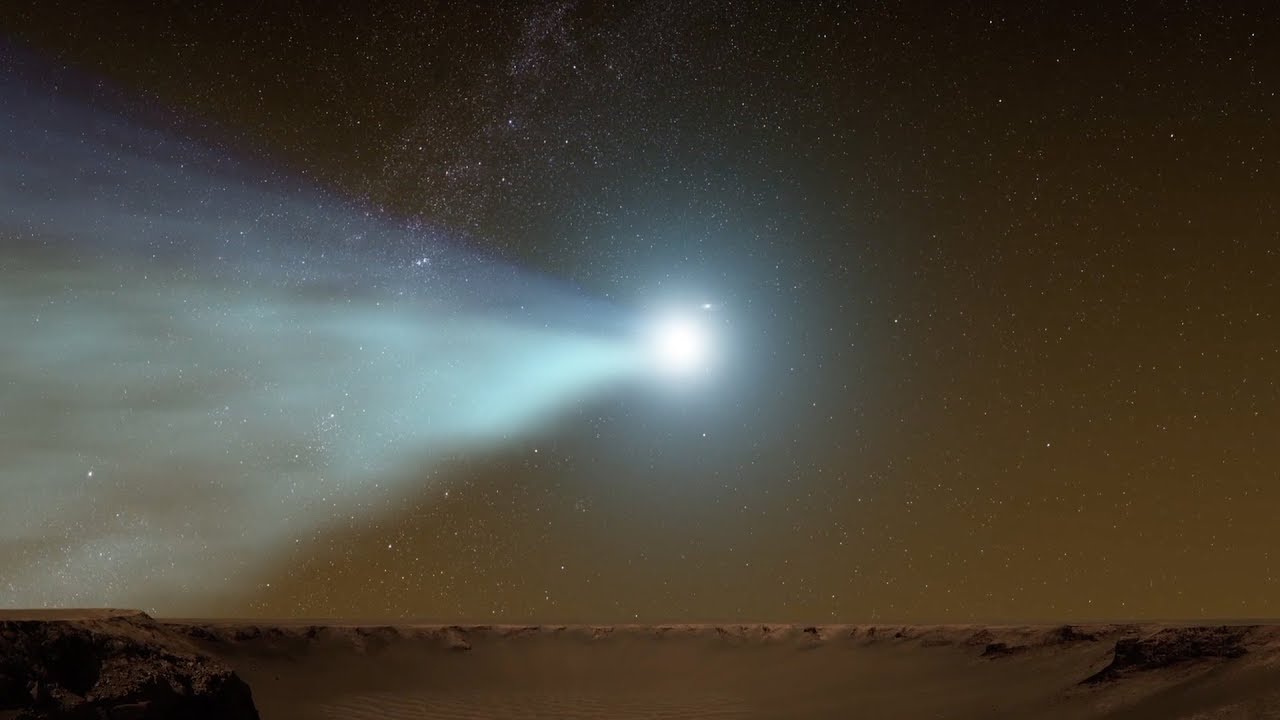This captivating image, which appears to be a painting or AI-generated, portrays a barren, lunar-like landscape under a surreal night sky. The ground, resembling a cratered and desolate surface, stretches beneath a sky filled with numerous stars and the faint outline of the Milky Way galaxy. Dominating the center is an intensely bright light source, perhaps meant to represent the Sun, despite the nighttime setting. This light emits a radiant, pyramid-shaped beam that pierces the darkness, illuminating the drab browns of the terrain and lending an otherworldly glow to the scene. The sky, tinged with shades of brown, complements the stark, almost alien atmosphere of this vivid and imaginative depiction.